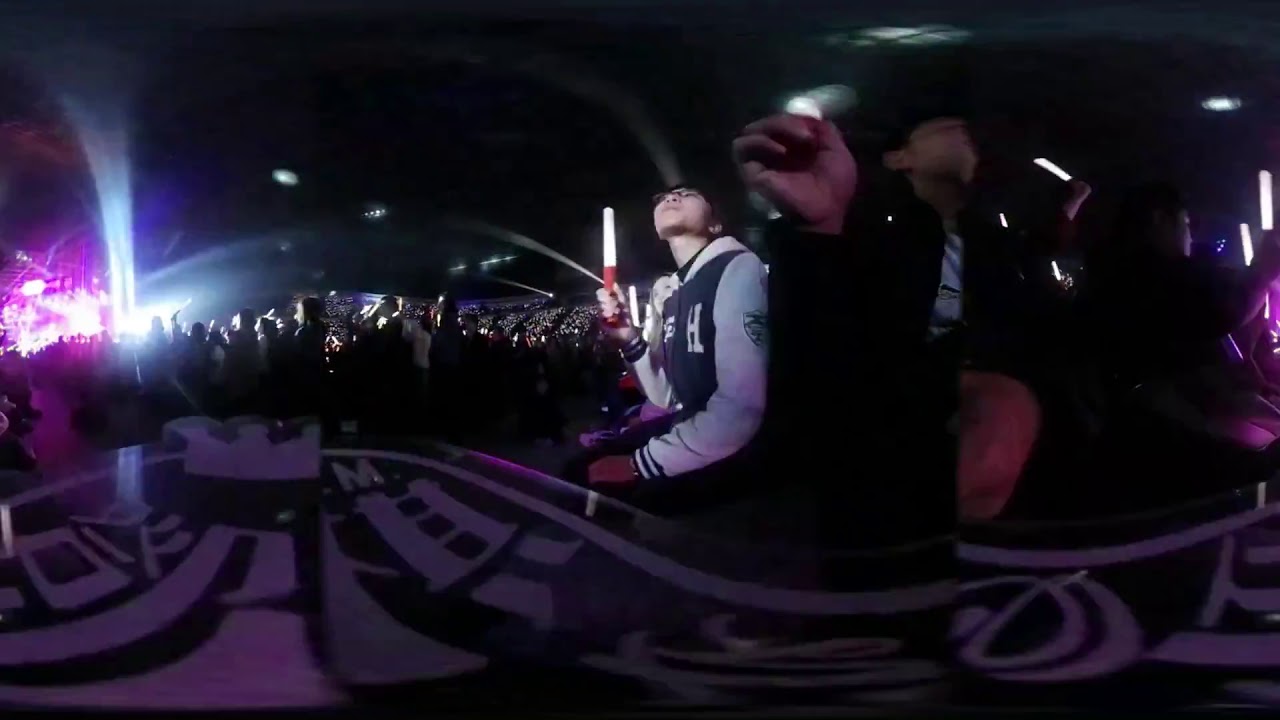The image depicts a dark, indoor concert venue or nightclub with a distinctive black and white contrast at the bottom and black at the top. Scattered throughout the scene are small white lights, contributing to the atmosphere. Front and center is a boy wearing a black and white jacket, his face illuminated by a bright white stick he is holding aloft. Behind him, a hand also extends into the frame clutching a similar light stick, silhouetted against the dim background. The left side of the image reveals a large crowd seen from behind, bathed in purple and white lights, and an ornate black and white image at the bottom. The venue features rows of angled seating, suggesting a concert hall, with a stage visible in the background, complete with drums and various lights casting swerving beams over the attendees. The stage lights dance around, adding to the dynamic and lively atmosphere. The floor and some seats appear to have a red hue, and across the center-left, more individuals can be seen lifting light sticks into the air. The bottom area of the picture includes a glossy surface with curved, possibly Asian characters, reflecting the surrounding lights.